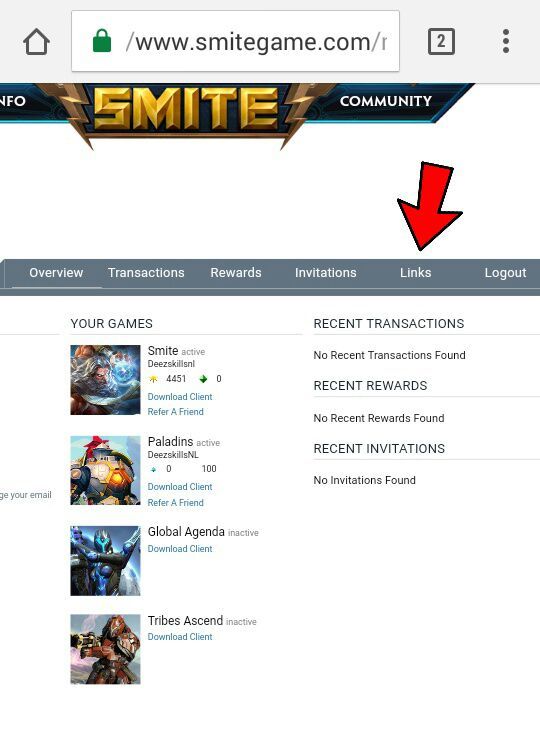Website Overview: HaasMyGame.com (x2)

**Primary Sections:**
- **Overview**
- **Transactions**
- **Rewards**
- **Invitations**
- **Radar**
- **Outputting of Links**
- **Logout**
- **New Games**
- **Smygg**
- **Keys**
- **Download Content** 
- **Refer a Friend**

**Games Featured:**
- Paladins
- Global Agenda

**Recent Activity:**
- **Transactions:** No recent transactions found.
- **Rewards:** No recent rewards found.
- **Invitations:** No recent invitations found.

**Highlighted Elements:**
- Yellow lettering and lightning bolts
- "Lightning bolts community" callout

**Navigation Summary:**
This comprehensive view includes sections for tracking and managing various aspects of the gaming experience, such as recent transactions, rewards, and invitations. The interface provides quick links for downloading game clients and referring friends to popular games like Paladins and Global Agenda. Features like "Smygg" and "transitsend" are also mentioned for further exploration. Digital elements and community-focused highlights enhance the website's interactive environment.